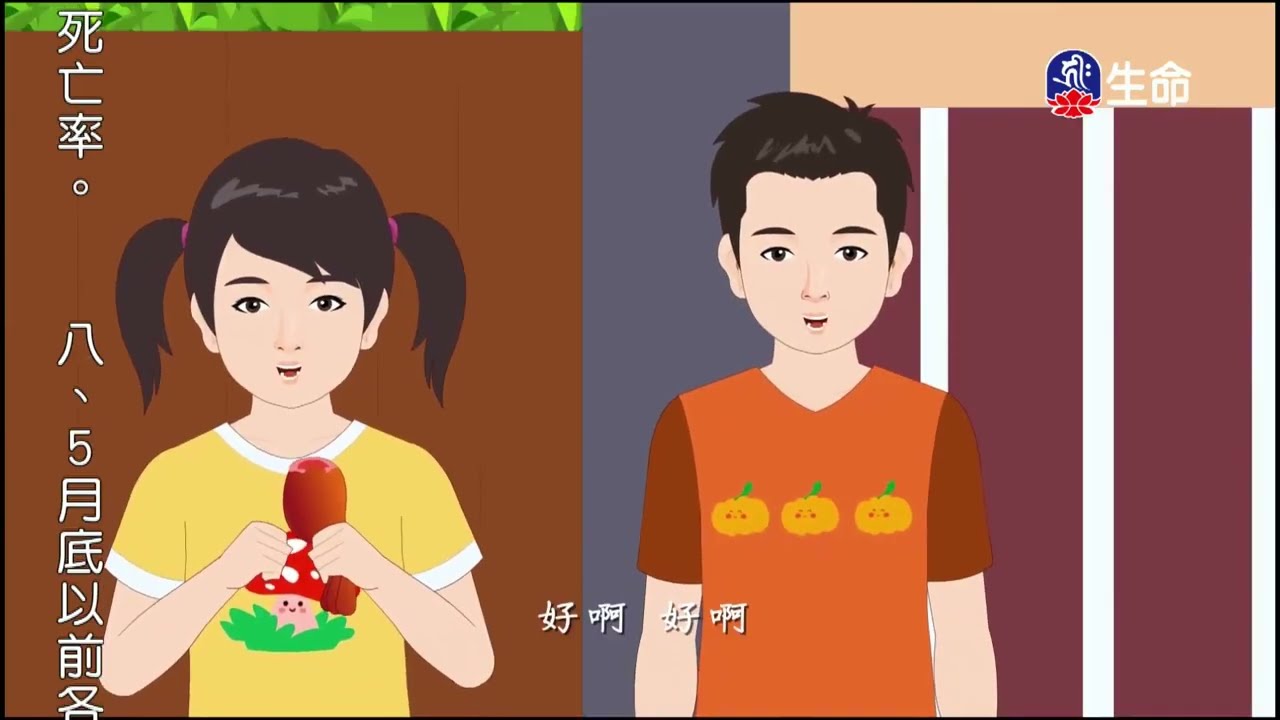In a brightly illustrated Asian cartoon scene, a young boy and girl stand in front of a wooden fence, suggesting an outdoor setting. The boy, taller with short dark hair, wears a short-sleeved orange shirt adorned with three pumpkins on the front. Beside him, the girl, who has her hair styled in pigtails, smiles happily, wearing a yellow short-sleeved shirt featuring a mushroom emerging from grass. There are Asian characters likely in Chinese script scattered throughout the image, with some positioned to the left of the girl and others at the bottom, resembling subtitles. The background includes a black house behind the boy, and a blue and red logo in the upper right corner of the screen. A number five also appears on the left side of the image.